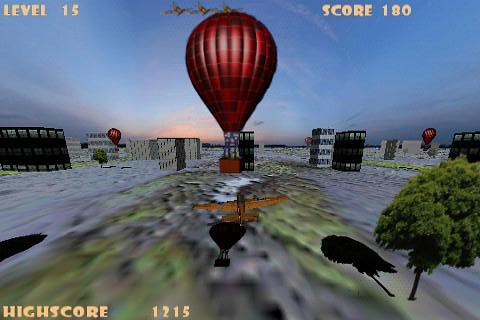This image is a computer-generated screenshot from a late 90s or early 2000s video game, characterized by its low-resolution, pixelated 3D graphics. In the upper left-hand corner, "level 15" is displayed in a yellow font, while the upper right-hand corner shows "score 180" in the same yellow font. The bottom left-hand corner reads "high score 1215." 

At the center of the image, a large red hot air balloon with a striped texture pattern dominates the scene. Alongside it, a small brown airplane appears to be the player's controllable object. The ground below features a blurry, pixelated mix of green and gray hues, also including the shadows of the tree and balloon. In the bottom right corner stands a small green tree.

The backdrop consists of several buildings scattered around, adding to the cityscape setting. There are additional hot air balloons in the distance, one on the left side of the frame and another near a large black structure or building. The sky is a gradient of blue and peach tones, suggesting a sunrise or sunset, with a hint of the sun visible in the center background.